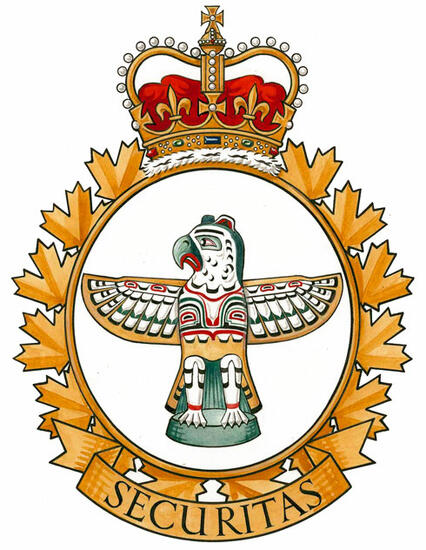The illustration depicts an official circular seal adorned with intricate designs and rich symbolism. At the top of the circle sits a royal crown with red velvet and ornate decorations, including pearls and an iron cross. Below the crown, encircling the seal, are golden maple leaves that contribute to the regal appearance. Central to the design is a white backdrop featuring an eagle with its wings spread, facing left. The eagle, reminiscent of Native American totem art, showcases a blend of gold, green, red, and white colors, with bold gold outlines and detailed decorative elements. The bird stands on a green pedestal, adding to its striking presence. At the bottom of the seal, a gold scripted banner elegantly displays the word "Securitas" in black font.